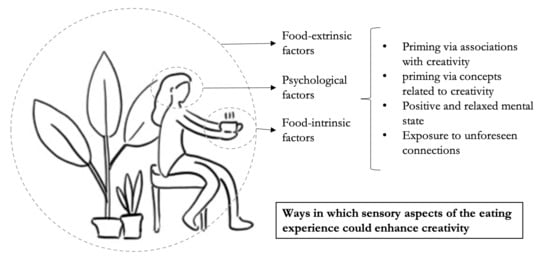The black-and-white diagram features a woman with long hair sitting on a stool, holding a steaming cup of hot beverage with both hands. Surrounding the woman, there's a dotted circular outline. Behind her are two potted plants: a tall plant with large, teardrop-shaped leaves and a shorter plant with three cactus-like leaves. Various arrows point from different parts of the image towards descriptive text on the right. The top arrow, pointing from a larger circle encompassing the entire scene, is labeled 'Food Extrinsic Factors.' The second arrow, pointing from around the woman's head, is labeled 'Psychological Factors,' and the third arrow, pointing from the cup, reads 'Food Intrinsic Factors.' To the right of these arrows, a bracket contains bullet points that list 'Priming via associations with creativity,' 'Priming via concepts related to creativity,' 'Positive and relaxed mental state,' and 'Exposure to unforeseen connections.' Below this detailed text, there is a black-outlined rectangular box stating, 'Ways in which sensory aspects of the eating experience could enhance creativity.' This detailed diagram is somewhat text-heavy, likely sourced from an informative textbook or instructional material.